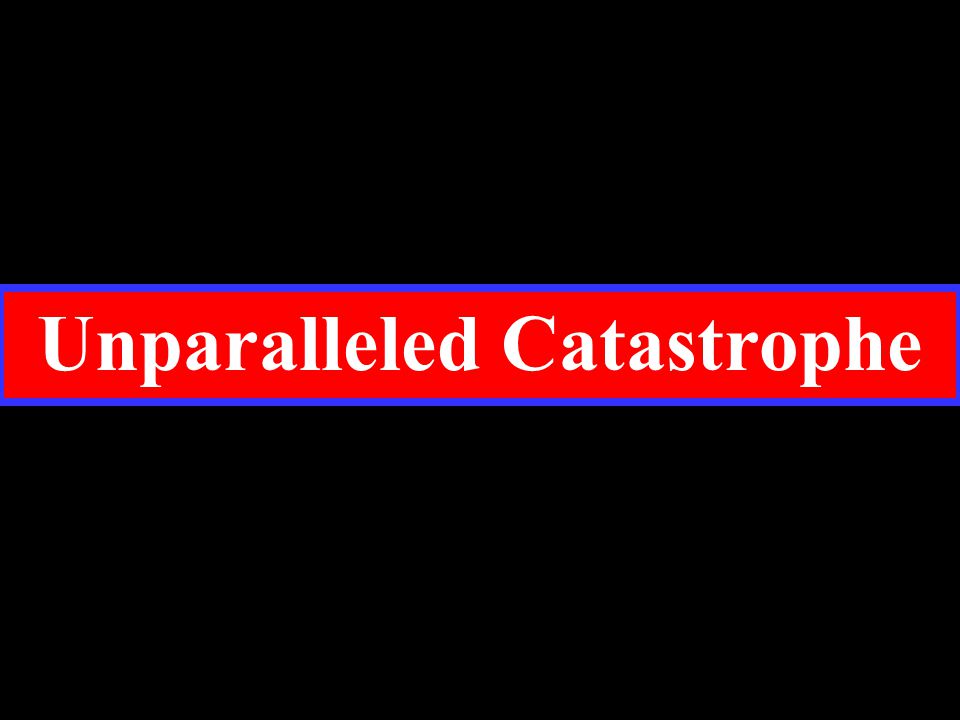This image features a stark black background, with a prominent red rectangular stripe running horizontally and centered both vertically and horizontally. The red stripe, which spans from the left center to the right center, is bordered by thin light blue lines on its top and bottom edges. In the center of the red stripe, in thick, easily legible white text, are the words "unparalleled catastrophe." The capitalization follows a specific pattern with "Unparalleled" having an uppercase 'U' and the rest in lowercase, while "Catastrophe" begins with an uppercase 'C' followed by lowercase letters. There is ample space on both sides of the words, ensuring that the text is centrally aligned and clearly visible against the contrasting colors.